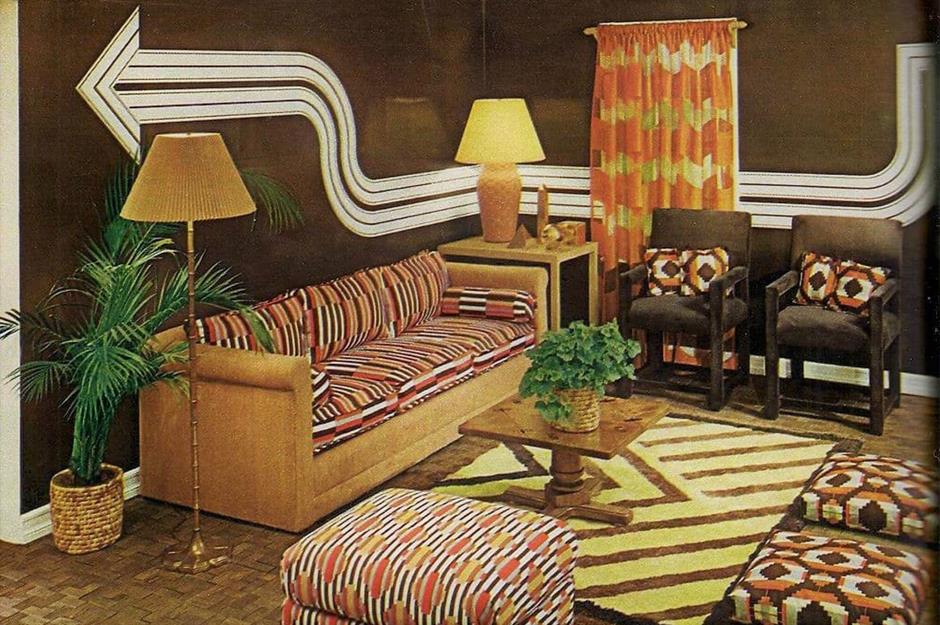This retro-inspired living room exudes a vintage vibe reminiscent of the 70s. The walls are painted a dark brown, adorned with a striking white arrow that spans from one end to the other, providing a dynamic and unique focal point. In the center of the room lies a zebra-like rug, with bold diagonal lines and V patterns in various shades of brown, adding to the eclectic decor. 

A long, three-seater sofa, featuring an orange hue and adorned with patterned cushions in shades of black, red, and white, is a central piece of furniture. Adjacent to the sofa is a hardwood or vinyl floor, and a square wooden coffee table with a potted plant as its centerpiece. Adding to the room's earthy tones are a couple of black chairs, each embellished with orange, white, and brown pillows.

A corner table with a stylish lamp sits next to the sofa, offering both function and aesthetic appeal. Another tall lamp stands nearby, enhancing the room's cozy atmosphere. Completing the scene is a tall, ficus-like palm tree in a woven brown basket, contributing to the lush, tropical feel of the space. The large windows are dressed with orange and green curtains, bringing a pop of color and tying the decor elements together harmoniously.